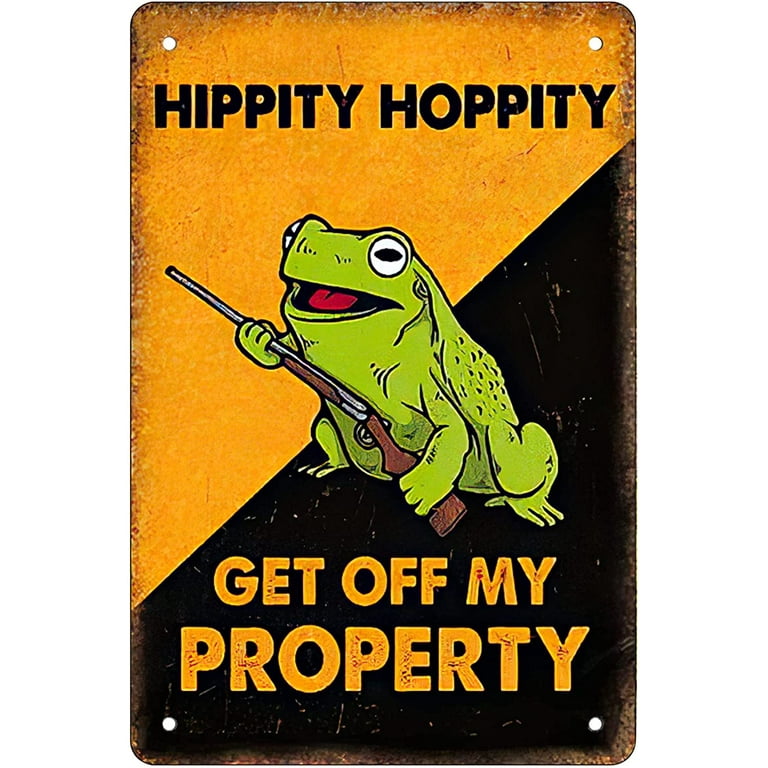The image is a vintage tin or metal sign featuring a detailed and somewhat humorous design. The background is split diagonally from the bottom left to the top right, with the top half in mustard yellow and the bottom half in black. At the top, written in black letters against the yellow backdrop, are the words "Hippity Hoppity," while the bottom half showcases the text "Get Off My Property" in mustard yellow letters on the black background.

In the center of the sign is a well-drawn green frog, depicted with a slightly open mouth and a red tongue. The frog, sitting hunched on its rear legs which are slightly spread apart, is holding a shotgun that faces the upper left side of the sign. This quirky and defensive posture adds to the humorous nature of the message. 

Surrounding the edges of the sign are signs of wear and rust, adding to its vintage aesthetic. Each corner of the sign has a punch hole, indicating it was once nailed to a surface. The green frog's sharp eyes—the black pupils within the white—enhance the lively and ironic feel of the image.